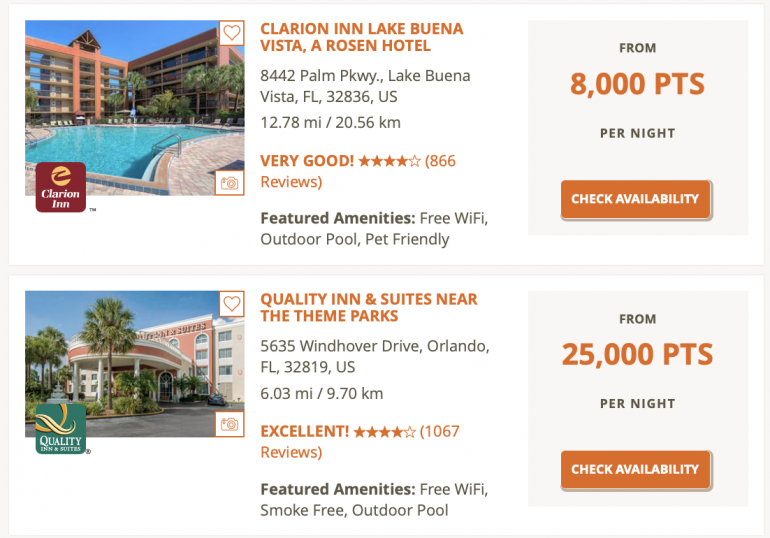The image depicts a travel or booking website featuring hotel accommodations. The page layout has a light gray background with large, predominantly white tiles occupying most of the central area. Each tile is approximately three-quarters white, with the right side displaying a light gray square box.

The first highlighted hotel is the **Clarion Inn Lake Buena Vista, a Rosen Hotel**, boasting a 4 out of 5 star rating. It offers stays starting at 8,000 points per night, with a button available to check its availability. 
Below it, the **Quality Inn and Suites Near the Theme Parks** is listed, also with a 4 out of 5 star rating, described as excellent. This hotel is priced from 25,000 points per night and includes a similar availability check button. 

Accompanying both listings on the left side are images of the respective hotels, providing a visual preview for potential guests.